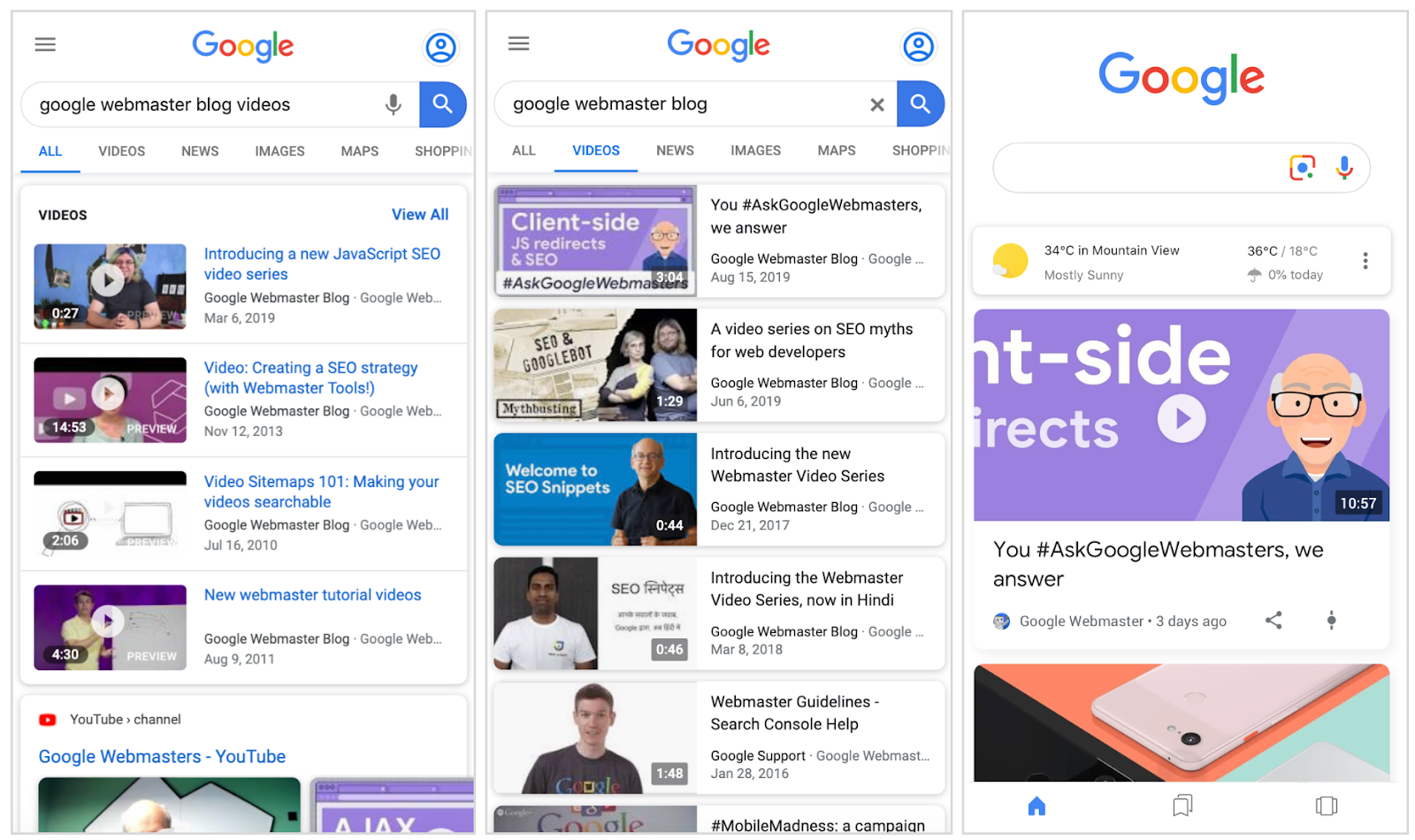**Detailed Descriptive Caption:**

The series of three screenshots showcases various elements of the Google Webmaster Blog video search interface and results. 

- **Screenshot 1:** At the top, it features the Google logo and a search query for "Google Webmaster Blog Video Search." The left-hand side of the interface displays a "Videos" filter, with a "View All" option on the right. Below the navigation bar are multiple video thumbnails:
  - The first video features a woman and is titled "Introducing a New JavaScript SEO Video Series."
  - The second video, which has a purple background, shows a woman and is titled "Creating an SEO Strategy with Webmaster Tools."
  - The third video displays an illustration of a TV set and is titled "Video Sitemaps 101: Making Your Videos Searchable."
  - The fourth video shows a woman against a purple background and is titled "New Webmaster Tutorial Videos."

- **Screenshot 2:** Also centered around a search for the Google Webmaster Blog, it displays additional video results:
  - The first video features a purple background with a cartoon bald character and is titled "You #AskGoogleWebmasters: A Video Series on SEO Myths for Web Developers," with a man and a woman introducing the content.
  - The second video shows a man in a black shirt against a blue background wearing a Google T-shirt and is related to "Webmaster Guidelines and Search Console Help."

- **Screenshot 3:** This final screenshot seems to be from a weather application or widget, showing the current weather in Mountain View, which is 34°C and mostly sunny with no rain forecasted. It also includes the video thumbnail of the "You #AskGoogleWebmasters" series with the purple background and cartoon characters, reiterating that "We answer your questions."

The detailed presentation of the search interface and video previews reveals a comprehensive guide for users seeking information on SEO, Webmaster tools, and related topics through a structured and visually consistent format on Google Webmaster Blog.